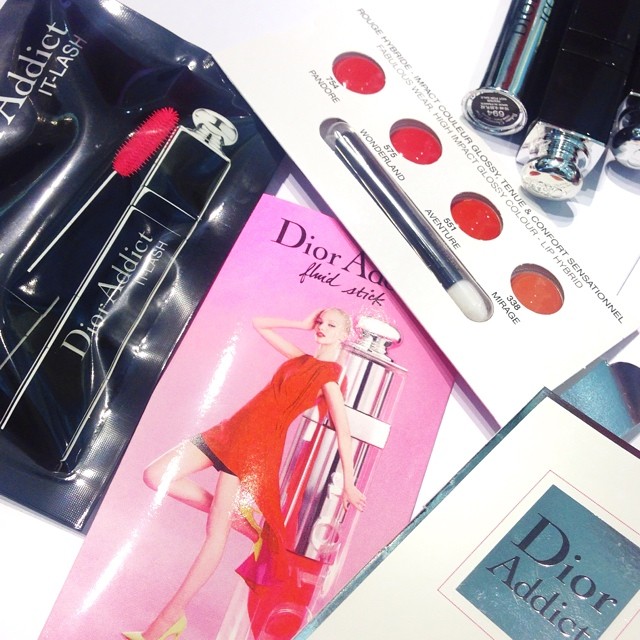This image is a detailed advertisement for Dior makeup products. In the upper left corner, there's a black bag containing three items: a black tube labeled "Dior Addict" in white, a mascara brush with a pink tip from the Dior Addict It-Lash collection, and a makeup palette with four distinct colors and an applicator. To the right of the bag, an open container showcases various colored makeup inserts. In the upper right corner, there are several tubes of makeup, possibly lipsticks, in different shades. Prominently displayed in the lower center, a pink package labeled "Dior Addict Fluid Stick" features an image of a woman in a flowing red dress, her right hand raised to her hair, set against a large makeup container. In the lower right, a blue box labeled "Dior Addict" is visible, further highlighting the range of Dior's beauty products. Overall, the table is filled with an array of Dior Addict cosmetics, emphasizing both eye and lip products.